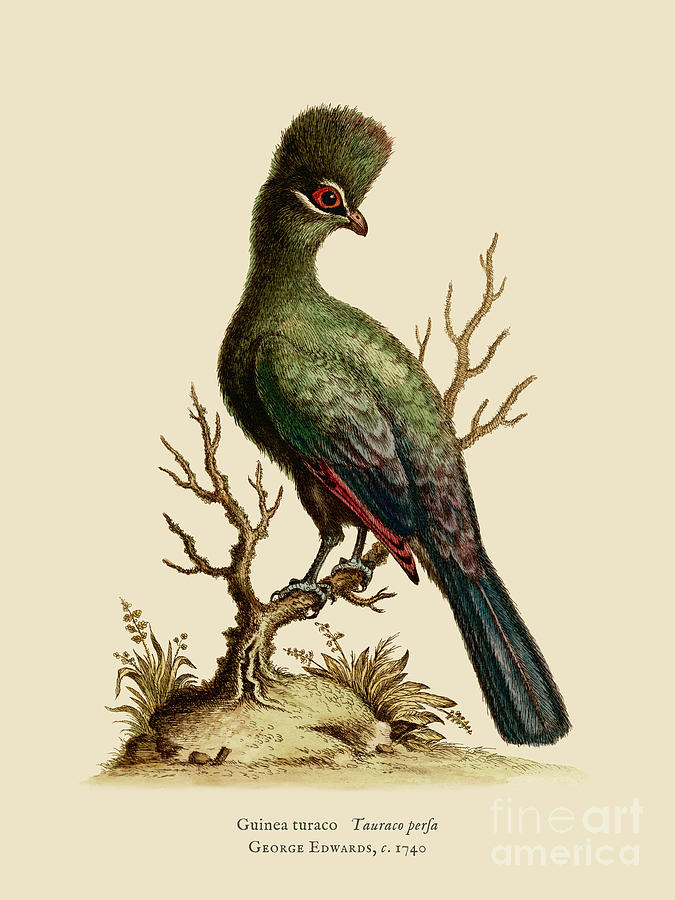This image is a detailed drawing by George Edwards circa 1740, showcased on light tan, possibly off-white or brown paper. It features a Guinea Turaco, also referred to as Turaco Perfa, with descriptive text at the bottom stating "Guinea Turaco, Turaco Perfa," along with "George Edwards, C. 1740" in italicized letters. The drawing captures a vivid outdoor scene with the bird perched on a Y-shaped tree branch. 

The Guinea Turaco has a striking green body, transitioning into brown feathers, and is distinguished by a dense tuft of upward-pointing feathers on its head, resembling a flat top haircut. The wings are beautifully adorned with orange edges, and it has a long black tail. The bird's head, which is turned to look downward from the top left to the bottom right, features a distinct red eye with a black pupil and a short, pointy yellow beak. The bird's grey legs are firmly gripping the branch, which is rooted in a tuft of grass with visible roots, surrounded by delicate flowers and plants on either side.

In the lower right corner of the image, the words "Fine Art America" appear prominently, indicating the source or publication of this artwork. This detailed and vibrant illustration combines anatomical precision with artistic elegance, capturing the Guinea Turaco in its natural habitat.